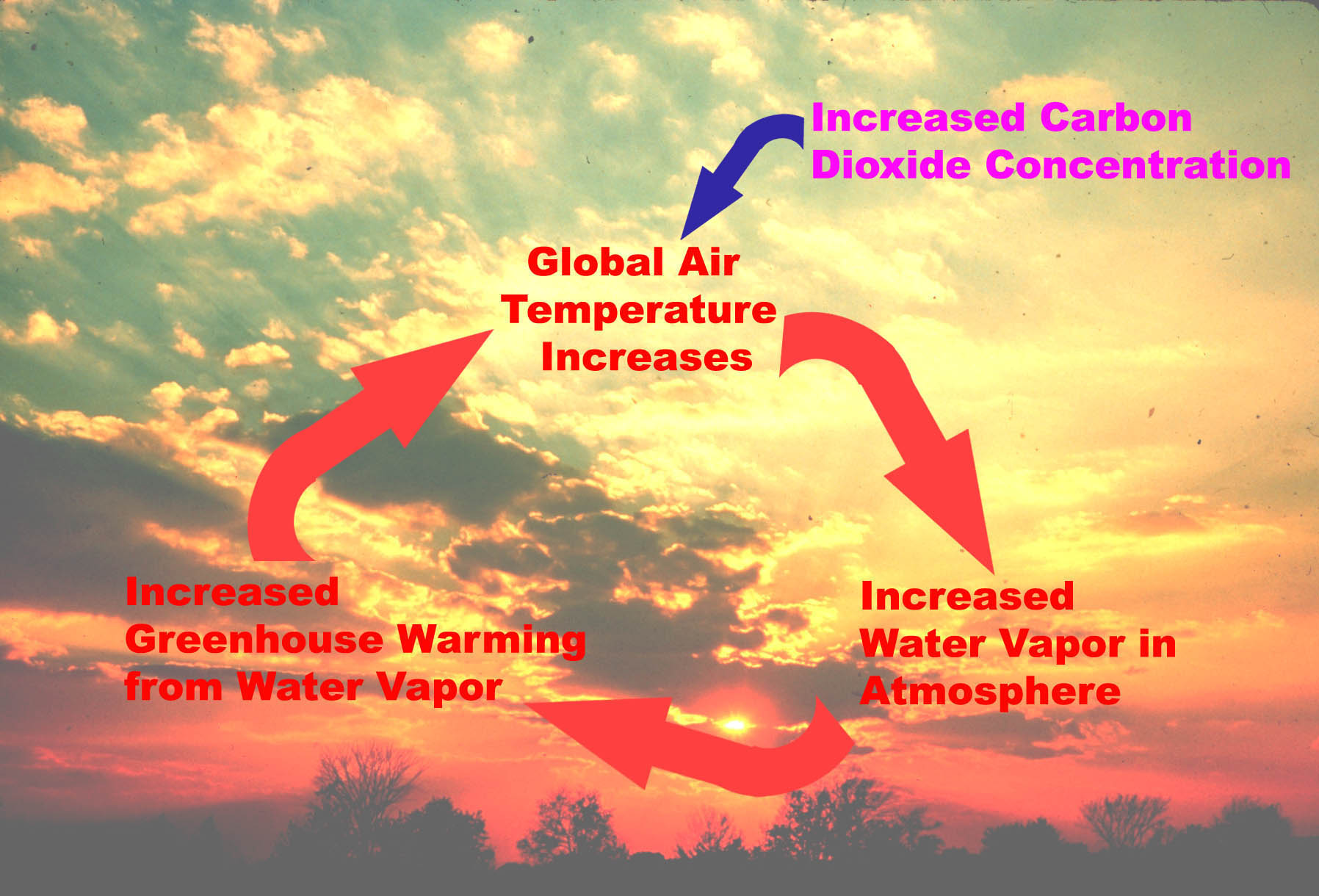The image is a horizontally aligned rectangular photograph of a vibrant, densely clouded sky with various colors. The top portion features a pretty blue sky with feathery, white clouds. The middle section blends darker gray clouds, while the bottom showcases a striking pink and yellow sunset, highlighted by the vibrant red hues near the horizon. The bottom edge of the image displays a slightly blurred silhouette of treetops.

Overlaying this dramatic sky are educational annotations with arrows forming a circular pattern, detailing the greenhouse gas effect. Centered in red text are the words "global air temperature increases," with a thick red arrow extending from the right towards the lower right, pointing to "increased water vapor in atmosphere." Another red arrow extends left from this point to "increased greenhouse warming from water vapor," which loops back with an upward right arrow to "global air temperature increases." Additionally, purple text in the top right corner reads "increased carbon dioxide concentration," connected by a blue arrow pointing down to "global air temperature increases," completing the circular illustration.